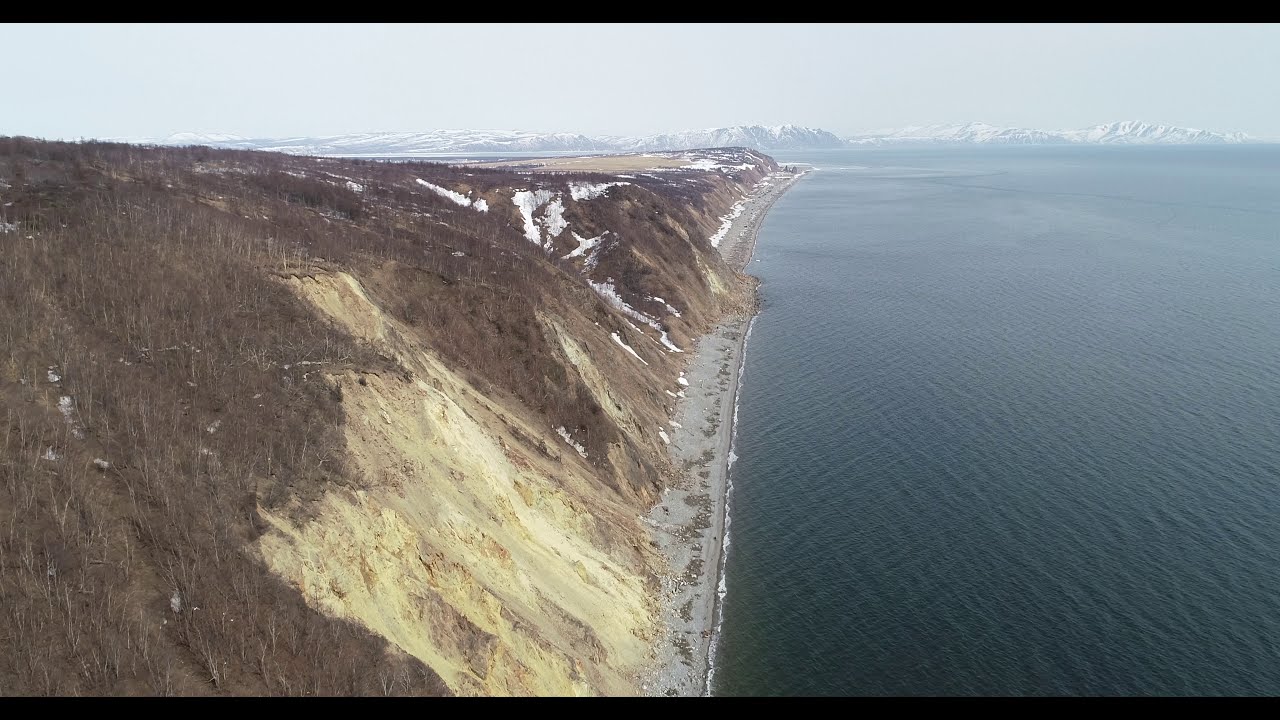The image presents a stunning aerial view of a rugged coastline where steep cliffs and hills meet a vast body of water. Dominating the left side, the cliffs and hills, which extend into the distance, showcase a striking palette from yellow to dark brown earth, capped with patches of brown foliage and small plants. A narrow line of gray beach, strewn with brown debris, separates the land from the water.

The dark, textured water occupies the center and right side of the image, appearing turbulent with ripples and waves that hint at its restless nature. The skyline is shrouded in a gray haze, contributing to the scene's somewhat somber mood. In the distant background, the faint outlines of snow-capped mountains or hills can be discerned through the mist.

Over to the horizon, there's a suggestion of far-off land with indistinct shapes that might be buildings or a tree line, though it's too hazy to tell for sure. This captivating landscape, with its contrasting elements of rocky terrain and deep, mysterious waters, evokes a sense of wilderness and remote beauty.